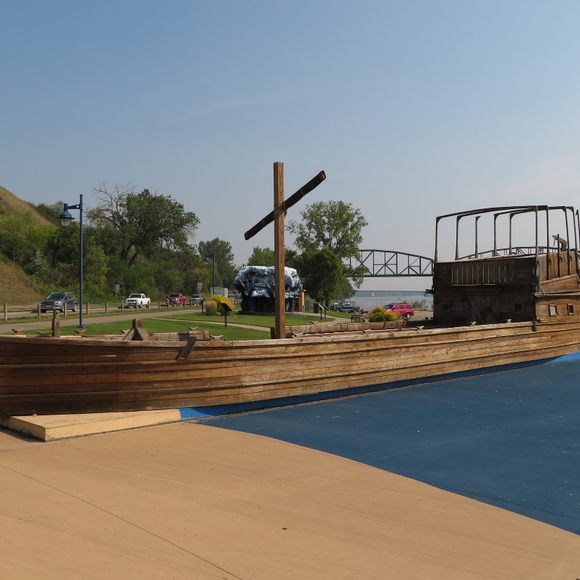The image depicts a large, intricately detailed wooden barge positioned on calm blue water, likely near a riverside park. The barge, with a medium stain, spans almost the entire width of the image. Dominating its design is a prominent wooden cross erected in the middle. The structure is long and flat with a taller hull at one end, featuring a framework suggesting a potential living or observation area. In the background, the scene opens up to a well-maintained landscape with grassy areas, trees, and a slight hill to the left. A bridge arcs gracefully over the water on the right, connecting the park to the road where several cars and trucks are parked. The sky above is a clear pale blue, enhancing the tranquil setting. The overall composition suggests a serene riverside area with a blend of natural beauty and manmade structures.